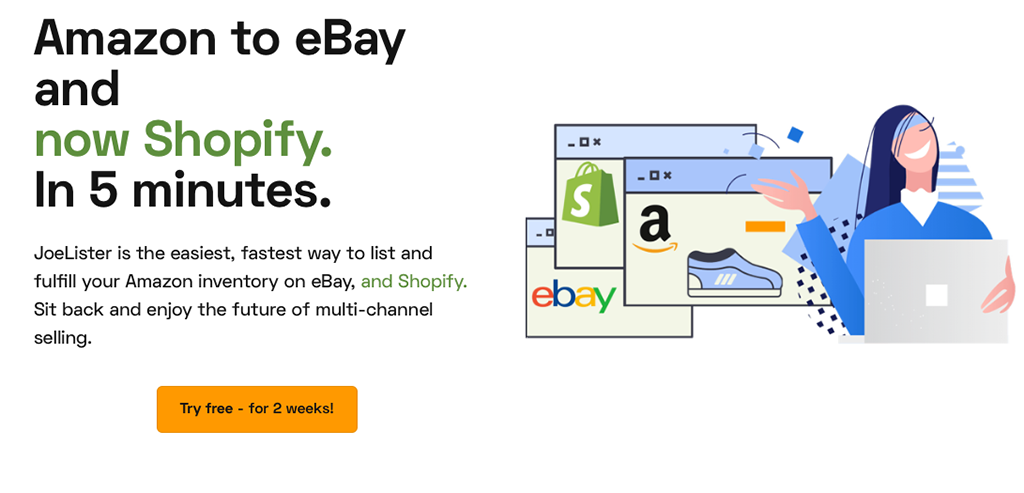The promotional image is divided into two sections. On the left side, a bold black text reads "Amazon to eBay," followed by a green text stating "now Shopify," and again in black, "in 5 minutes." Below this, in smaller writing, it says, "Joe Lister is the easiest, fastest way to list and fulfill your Amazon inventory on eBay," then in green, "and Shopify," and back in black, "Sit back and enjoy the future of multi-channel selling." At the bottom, there's an orange rectangular button with rounded corners that reads, "Try Free for 2 Weeks."

On the right side of the image, there is a visual depiction of a woman using a laptop. She appears to be tossing two blue squares, one light and one dark, into the air. Additionally, there is a detailed image featuring a blue rectangle with a picture of a shoe, accompanied by the Amazon logo and an orange triangle. Behind this, part of a green shopping bag with an "S" on it is visible, as well as a partial view of the word "eBay."